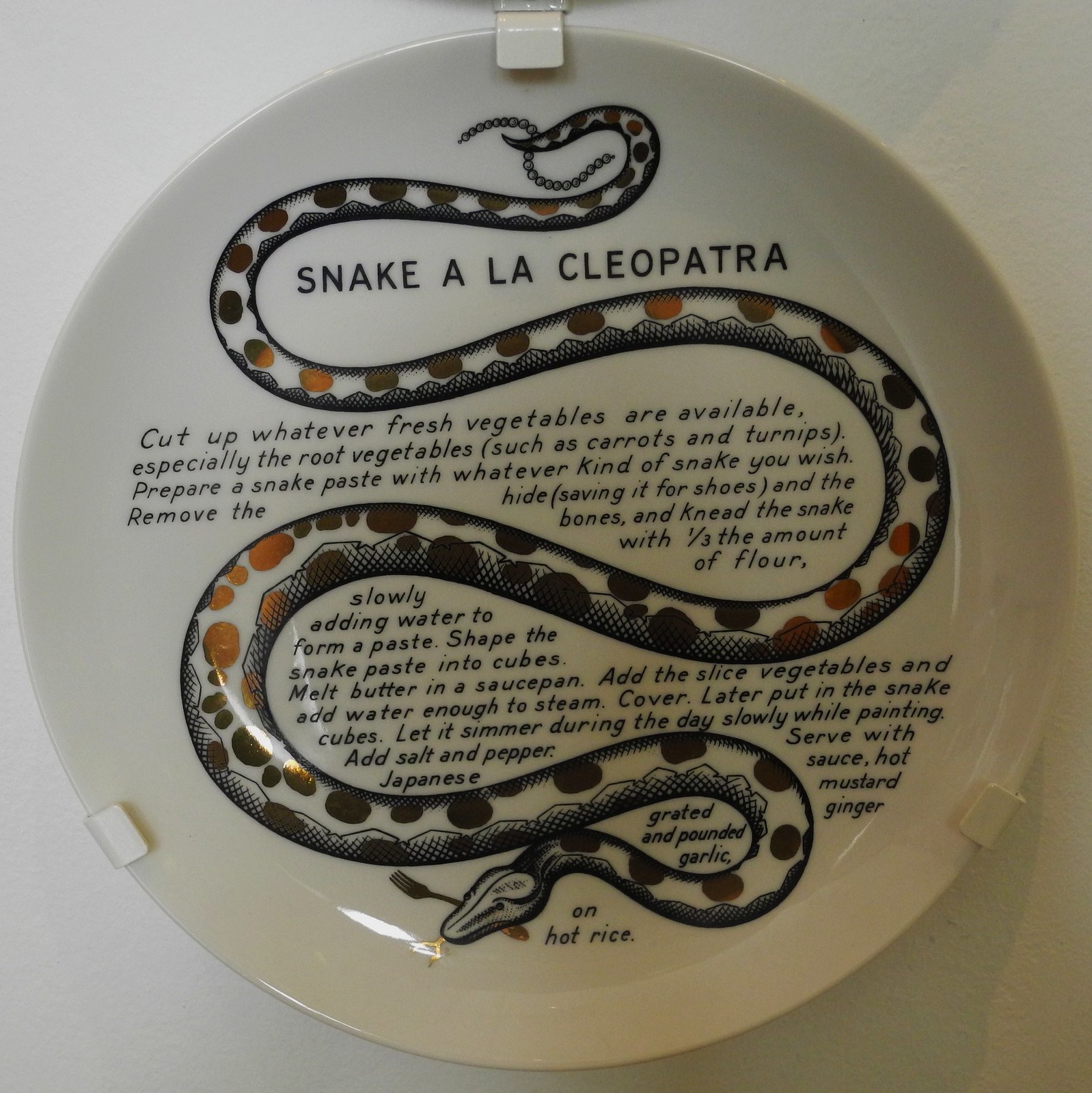The image features a decorative white plate, framed with a black border and mounted on the wall with brackets. Dominating the design is a detailed depiction of a snake that zigzags and spirals from the top to the bottom of the plate. The snake's body is white, highlighted with black and gold circles, and brown spots. Across the top, in bold black font, the plate reads "Snake à la Cleopatra," with the snake's head positioned at the bottom, resting on a small gold fork. Embedded within the intricate snake design are detailed instructions on how to prepare a dish using snake meat. The text suggests chopping fresh vegetables, particularly root ones like carrots and turnips, creating a snake paste with snake meat and flour, and simmering the mixture slowly while incorporating various seasonings and sauces to serve with hot rice.